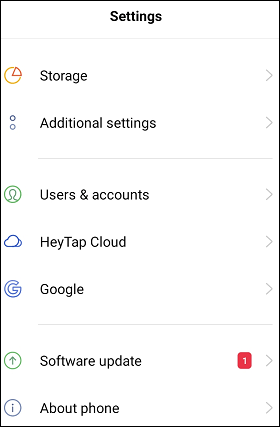This image is a screenshot from my website, showcasing the settings menu interface. The central focus is a vertically-oriented rectangle with a thin black border and a white background. At the top, in bold black print, is the title "Settings" with a capital 'S'. Below this heading, the menu is organized with icons aligned on the left side, accompanied by text items listed in black with each word capitalized.

The first menu item is "Storage," followed by "Additional Settings." Next are "Users and Accounts," then "Heytap Cloud" (where "Heytap" is styled as one word with a capital 'H' and 'T'). Following this is "Google," and then a horizontal line divider. Below the divider, the options continue with "Software Update" and "About Phone."

To the right of "Software Update," there is a small red square containing the number '1' in white text, indicating a notification or update. Each menu item is accompanied by a right-facing arrow on the far right side, indicating that selecting the item will lead to a sub-menu or additional details.